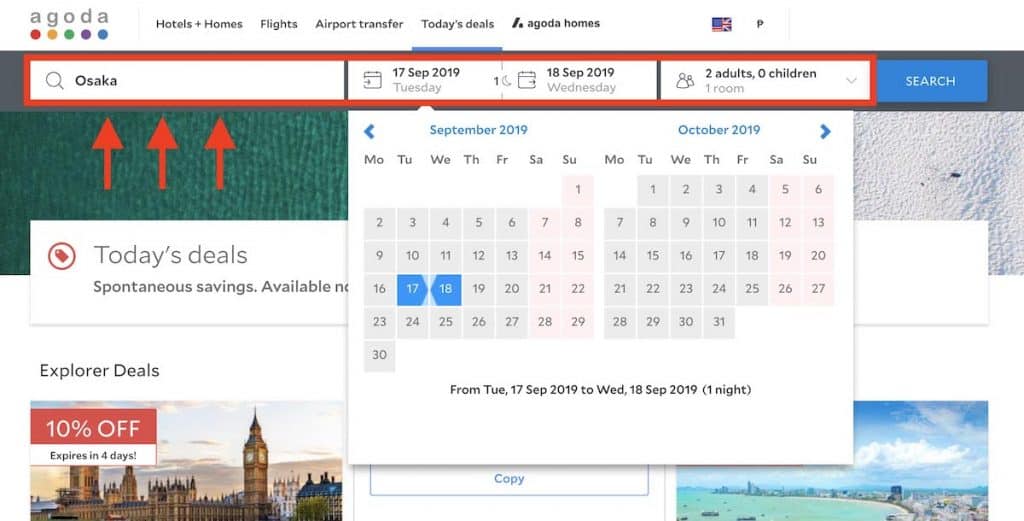This image is a screenshot of a booking website interface. At the top, against a white background, there are five small colored circles, each paired with gray text above them. From left to right, the circles are red labeled 'A,' yellow labeled 'G,' green labeled 'O,' purple labeled 'D,' and blue labeled 'A.' To the right of these circles, the text reads 'Hotels and Homes,' 'Flights,' 'Airport Transfer,' and 'Today's Deals,' with 'Agoda Homes' underlined in blue.

Below this header, there is a visualization featuring half of the American flag on the left and half of the UK flag on the right, indicating a choice of language or region.

Underneath the flags are search boxes and bars. The leftmost search bar, outlined in red, is white with a magnifying glass icon on the left side. Inside this search bar, black text reads "Osaka." Adjacent to this is the date selector showing 'September 17, 2019, Tuesday' and 'September 18, 2019, Wednesday.' Further to the right, it displays 'Two adults, zero children, one room,' with a dropdown option indicated.

Beneath these inputs, an open calendar for September and October 2019 is displayed. The dates 'September 17' and '18' are highlighted in blue, indicating the selected dates. On the left side of this section, against a dark green background, there are three red arrows pointing upwards toward the search bar above, emphasizing it.